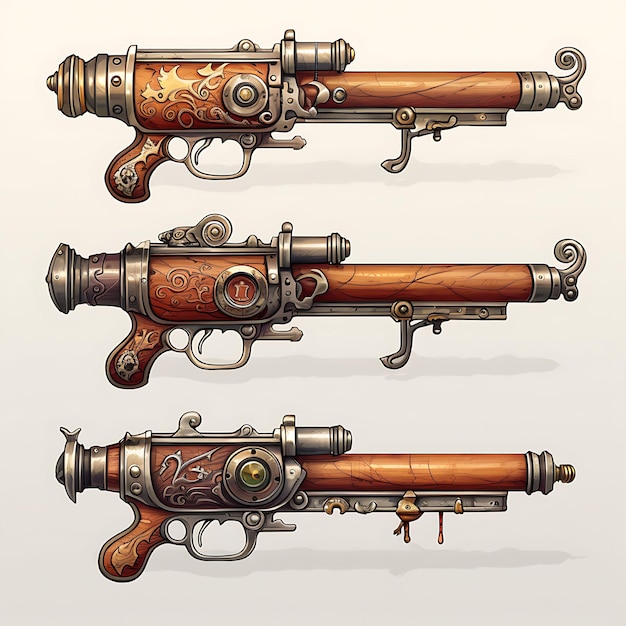The image displays a meticulously detailed drawing of three antique-style muskets, each with distinct steampunk influences, set against a light gray to tan or cream-hued background. The layout appears nearly square, lending an elegant symmetry to the arrangement. Each musket showcases a harmonious blend of light brown wood and silvery metal elements, yet they differ in their decorative details and structural components.

The handles of all three guns exhibit unique designs near the trigger area, highlighted by artistic variations. The barrels, though similar in overall shape and size, each feature distinctive ends: the top musket has a silver cap with a curled metal section, the middle one sports a round knob, and the bottom musket is adorned with a bulbous extension resembling a knife. Each trigger guard is crafted from brown metal, with a graceful curve marking the trigger line. The subtle play of shadows behind each gun further accentuates their intricate designs, suggesting they may be machine-generated with a touch of hand-drawn artistry. This image exquisitely captures the craftsmanship and diverse artistic flourishes of what appears to be creations from the same imaginative gunsmith.